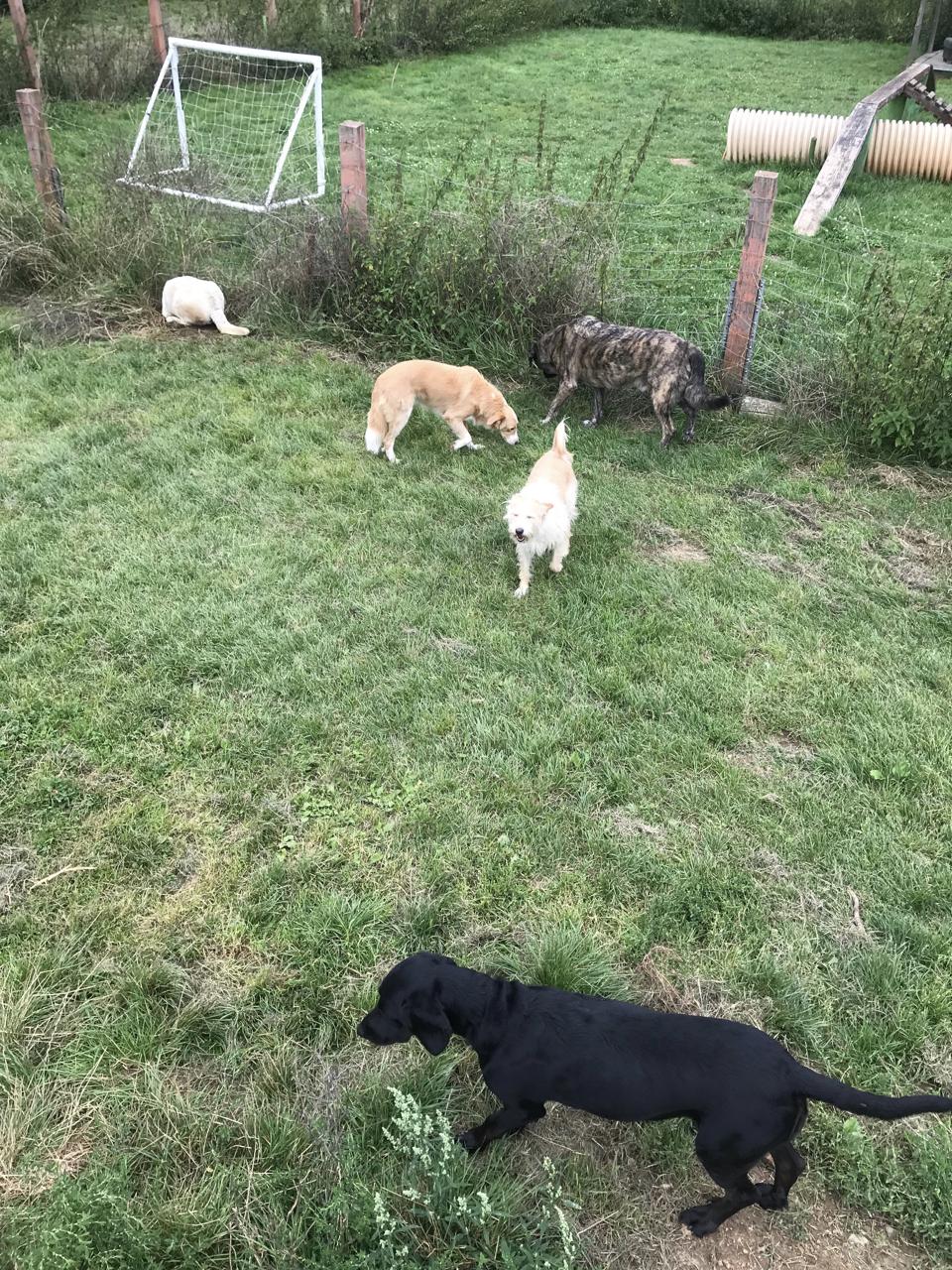This vibrant color photograph captures a lively moment featuring five dogs in a grassy yard. The backdrop is predominantly green grass, interspersed with patches of drier, yellowing areas. On the left side of the image, a white dog with a light tan tail digs energetically under a fence made of wooden, reddish posts interspersed with bare, tall bushes. The center of the scene is dominated by three dogs of various breeds: a brindle-coated dog stands close to the small wooden fence near the middle, flanked by two tan dogs, one sniffing the ground and the other standing nearby. To the right, a young black Labrador or possibly a black hound is seen sniffing the grass. In the distance, to the top left of the photograph, a white soccer goal with light-colored netting is visible, adding a playful element to the setting. Adjacent to this, on the top right, lies a large circular pipe, perhaps for some construction purpose, subtly indicating the multi-functional nature of the yard.